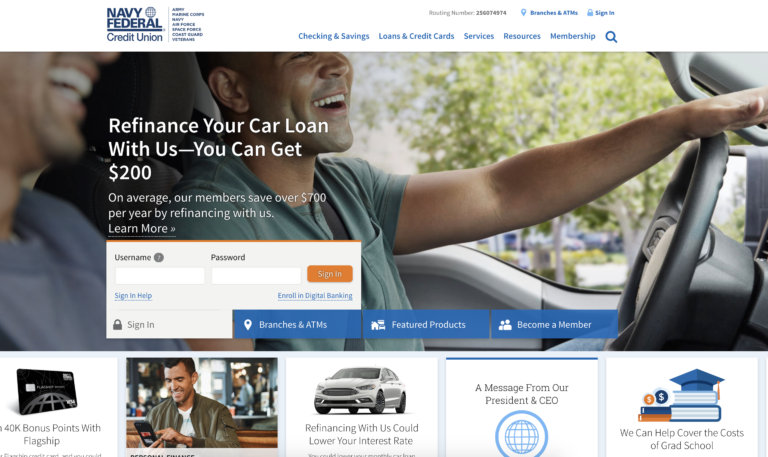The webpage features a comprehensive and user-friendly design catering to Navy Federal Credit Union members. In the top left corner, the Navy Federal Credit Union logo is prominently displayed. Centered towards the top are links to various branches of the military: Army, Marine Corps, Navy, Air Force, Space Force, as well as options for Coast Guard and Veterans.

On the top right, essential links for Routing Number, Branches and ATMs, and Sign In are easily accessible. The webpage's header uses white space for clear navigation, but there is a color scheme of blue text against a white background, which might not be to everyone's liking.

On the right-hand side, there's a section for Services, Resources, and Membership, each providing detailed information. A blue magnifying glass icon for search functionality is positioned on the far right.

In the center of the page, there is a large image of a smiling man gesturing towards his car. Overlaying this image is an enticing offer: "Refinance your car loan with us, you can get $200 on average, and save over $700 per year by refinancing with us."

Below the image, there are fields for Username, Password, and a Sign-in button, along with additional links for Branches and ATMs, Featured Products, and Become a Member, all housed within a blue rectangular overlay.

At the very bottom, five distinct boxes span from left to right, providing various messages, website functionalities, and notifications, rounding out the homepage with a wealth of resources and information for users.